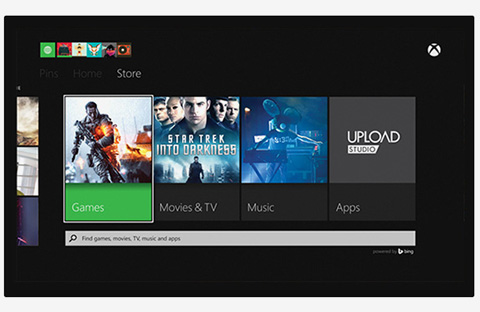The image depicts a predominantly black screen with subtle detailing. Encasing the screen at the top and bottom are thin, light gray borders. Against this black backdrop, six small icons are evenly spaced at the top of the image, each icon housed within its own square. 

1. The first icon is green with a centered circle.
2. The second icon is red, featuring a black image.
3. The third icon is gray, displaying a yellow cartoon character.
4. The fourth icon is turquoise blue, also featuring a cartoon character.
5. The fifth icon is gray, depicting what appears to be a monkey.
6. The sixth icon is black with an orange center.

Moving down the screen, the left side displays partial graphics. Centrally, there are four distinct sections:

1. The first section is labeled "Games" and shows a dynamic video game in action.
2. The second section is titled "Movies & TV" and highlights a scene from "Star Trek Into Darkness."
3. The third section is dedicated to "Music."
4. The fourth section pertains to "Apps," specifically featuring "Upload Studio."

At the bottom of the screen, a banner displays a search engine bar adorned with a magnifying glass icon alongside a prompt that reads, "Find games, movies, TV, music, and apps."